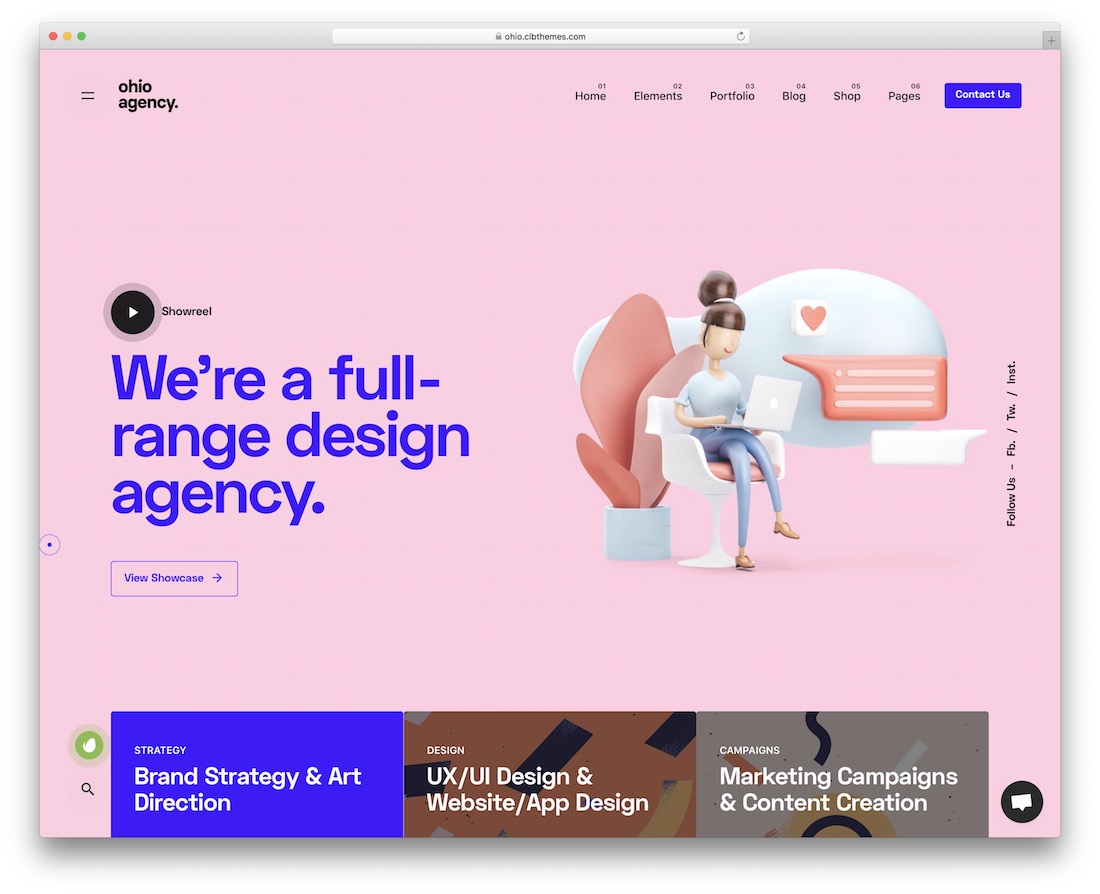The image showcases the homepage of the OIO Agency's website, prominently displayed with its logo in the top left corner. The website's navigation bar spans across the top, providing options to explore Home, Elements, Portfolio, Blog, Shop, and Pages, along with a distinct blue "Contact Us" button on the top right.

In the center, slightly to the right, there is an illustrated image of a woman seated on a chair, with plants adorning the background. To the left of this image, set in blue text, is the declaration, "We're a full-range design agency." Above this text, a small button is available for playing a video titled "Show Reel." Below the text, another button invites users to "View Showcase."

Towards the lower section of the screen, three rectangular sections present concise overviews of the agency's core services. The first rectangle, labeled "Strategy," highlights their expertise in brand strategy and art direction. The second rectangle, "Design," enumerates capabilities in UX/UI design, website creation, and app design. The third rectangle, "Campaigns," details their proficiency in marketing campaigns and content creation. Design patterns provide a visually appealing background for these sections, enhancing the overall aesthetic of the website.